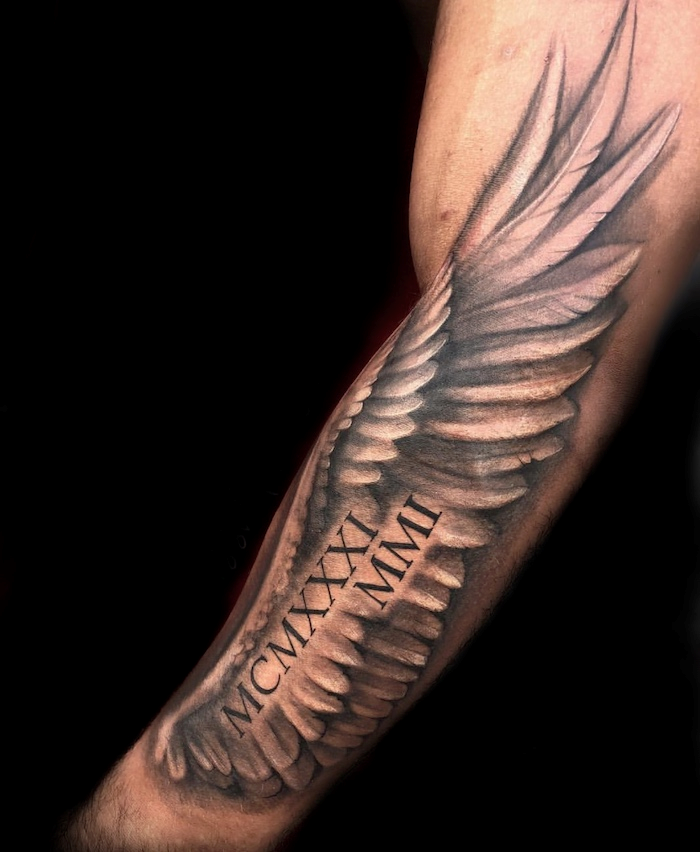This close-up photographic image captures the left arm of a white man, showcasing an intricate tattoo. The tattoo, an artistic depiction of an eagle's wing, extends from the base of the shoulder down towards just above the wrist. The wing's feathers are rendered in varying shades of gray and brown, with the largest feathers prominently displayed on the bicep and smaller ones tapering down around the elbow. Roman numerals, MCMXXI and MMI, are inscribed below the wing, likely denoting significant dates. The arm is set against a solid black background, either from a black t-shirt or curtain, emphasizing the tattoo's vibrant details. Notably, a bulging vein is visible on the bicep, adding to the realism and texture of the photograph.